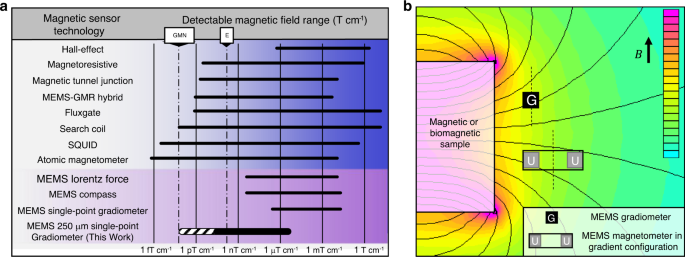The image is an information graphic about magnetic sensor technology, divided into two distinct sections labeled A and B. Section A, on the left, features a detailed chart below the heading "Magnetic Sensor Technology," listing various types of sensors: Hall effect, magnetoresistive, magnetic tunnel junction, MEMS-GMR hybrid, flux gate, search coil, SQUID, atomic magnetometer, MEMS Lorentz force, MEMS compass, MEMS single point gradiometer, and MEMS 250 single point gradiometer. Alongside these sensors is a chart titled "Detectable Magnetic Field Range," displaying numerical values and lines indicating their respective field ranges. Each sensor's range is depicted with varying line lengths, emphasizing the sensitivity differences among the technologies.

Section B, to the right, showcases a multicolored chart on a predominantly green background transitioning from blue at the bottom to pink at the top, denoting increasing measurement values. This section discusses "Magnetic or Biomagnetic Sample," indicating waveforms and measurements focused on MEMS gradiometers and MEMS magnetometers in gradient configuration. The chart features a color scale from blue through green, yellow, orange, and pink, with pink representing the highest values. Additional annotations include a legend clarifying the labels G (MEMS gradiometer) and U (MEMS magnetometer) to delineate the equipment used for measuring the samples.